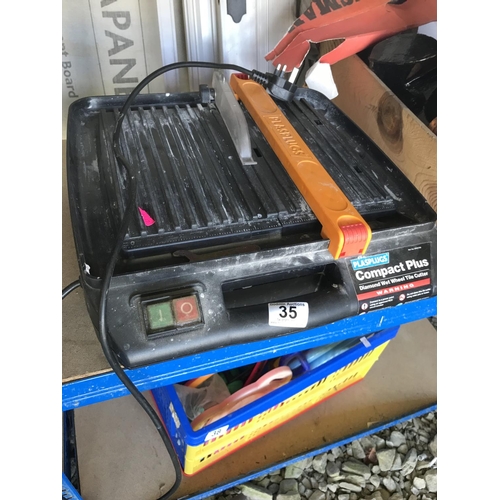The image depicts a compact construction saw stationed outdoors on a gray gravel surface. The main body of the machine is encased in black plastic, with a yellow handle and an additional silver handle on the top. The front of the machine features green and red buttons, the green being square and labeled as the power-on button, and the red being round and marked as the power-off button. A black wire extends from the left side, and a conspicuous yellow bar runs from the back to the front, aligned with a black part presumed to be the machine's primary cutting component.

Prominently, on the right side of the machine, there's a label that reads "PLASPLUGS" above a green background with white text, followed by a larger black label stating "Compact Plus." Beneath this, in smaller, difficult-to-read text, it mentions "Diamond Wet," accompanied by a visible warning sign below. The machine appears to have a base with ridges on the top, reminiscent of a drainage tray, and a plastic guard presumed to safeguard the saw blade. The scene is cluttered, with pieces of wood or drywall scattered around, and below the machine, there is a yellow basket with a blue handle containing various tools. Notably, the top of the machine features a flesh-toned, computer-generated hand hovering above it.